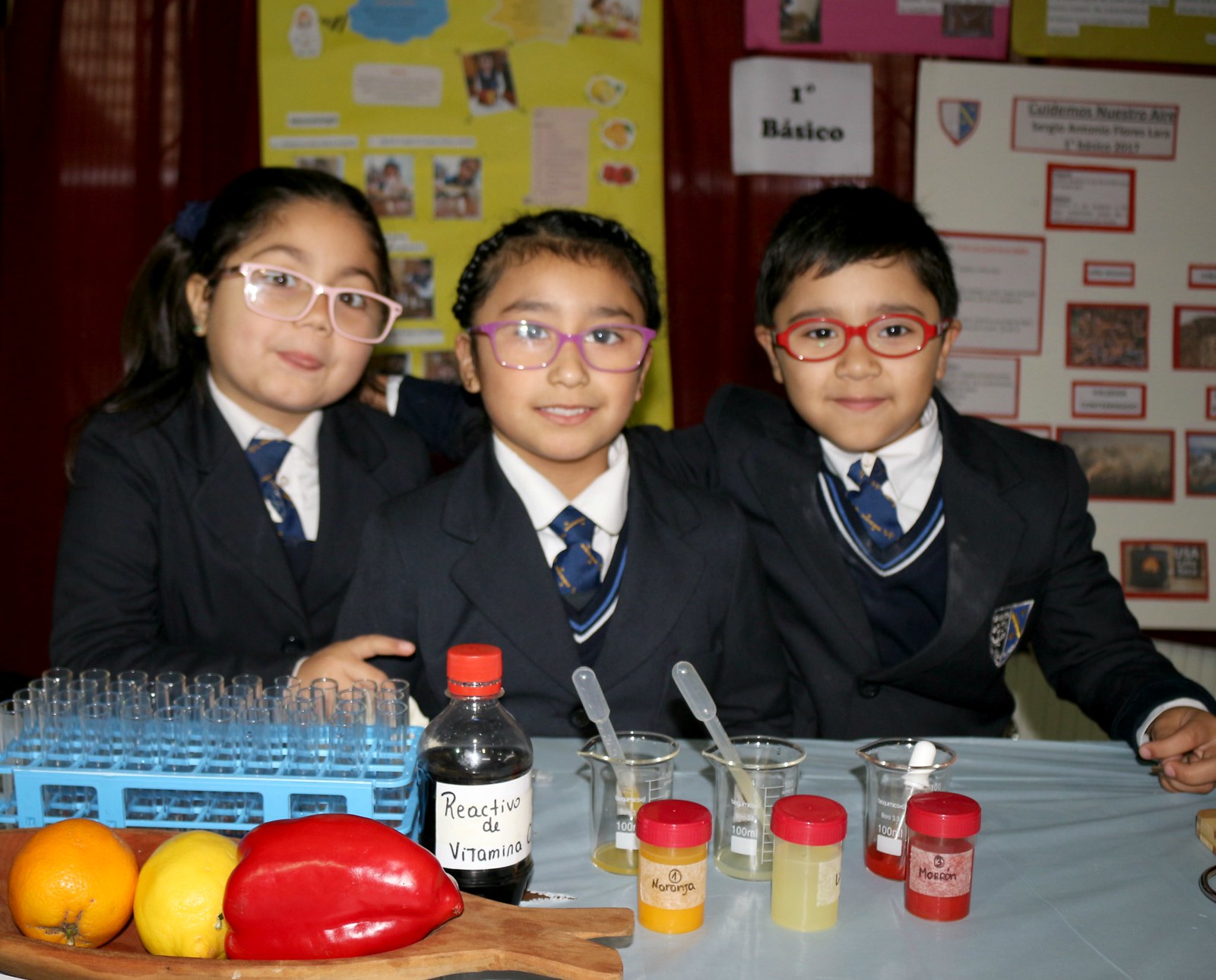The image captures three smiling children seated at a table in a bright, school setting, with colorful science posters mounted on the wall behind them. They are all dressed in matching school uniforms consisting of a white collared shirt, blue tie, and a black blazer. Each child wears glasses; the girl on the left sports light pink frames, the center girl has braided hair and wears blue and purple glasses, and the boy on the right has red glasses.

In front of them on the table are several scientific items: clear glass test tubes, a bottle labeled "Reactivo D Vitamins," small clear bottles containing orange, yellow, and red liquids, and beakers behind each of these bottles, each with a pipette. Additionally, there is a wooden tray in the bottom left corner holding an orange, a lemon, and a red bell pepper. The overall scene is bright and lively, accentuated by the light and the children's evident interest in the experiment.